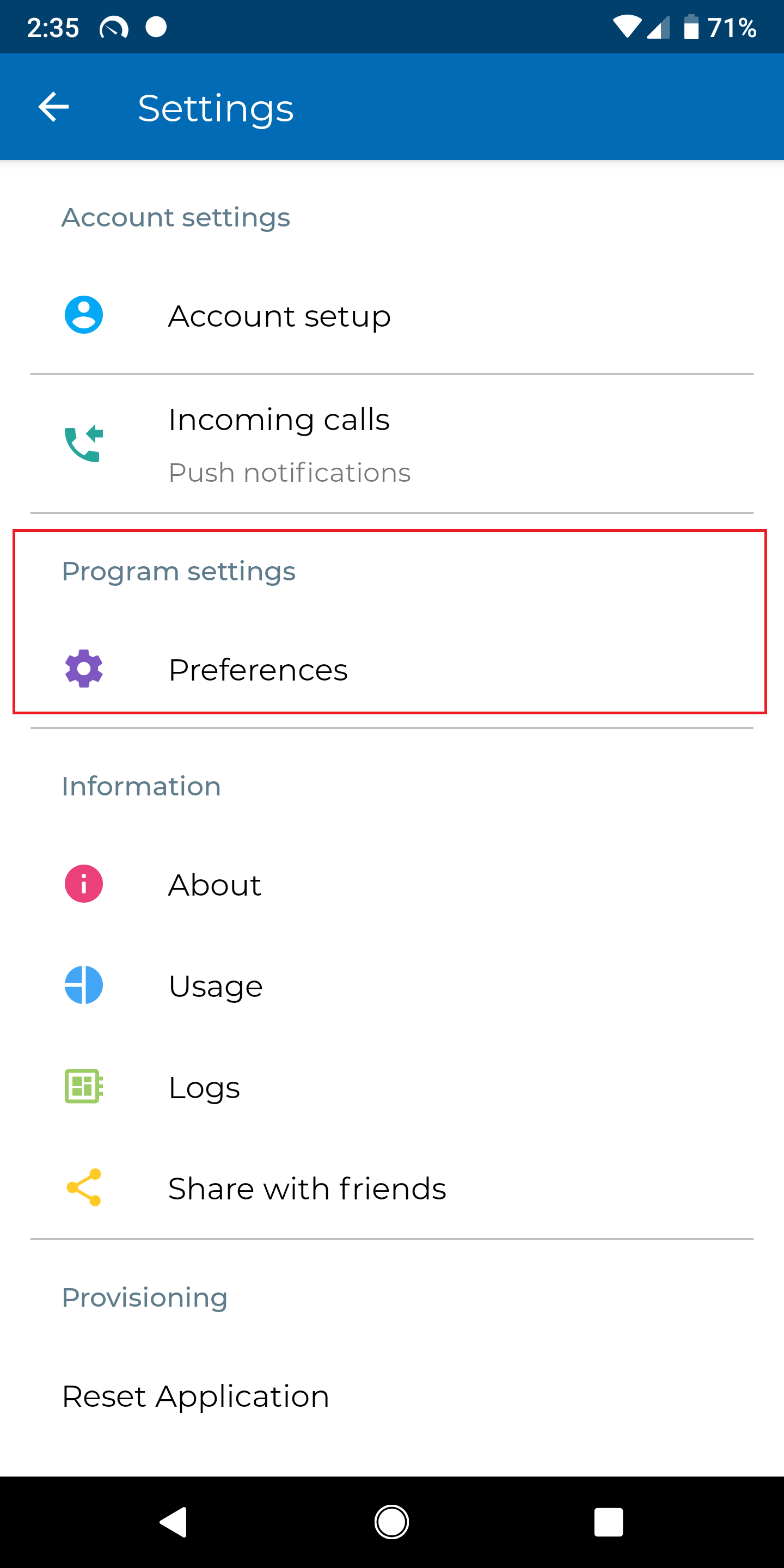The image is a screenshot from a smartphone displaying the settings interface. The top section is highlighted in a blue rectangle, indicating that the user is in the 'Settings' section of the phone. The primary background is composed of various shades of blue, with additional colors such as green, pink, yellow, white, purple, red, and black permeating through different icons and text.

At the top, in the blue section, it clearly states 'Settings,' and just below that is a red rectangular outline emphasizing 'Program Settings and Preferences.' The text within this section is written in black, while the icons are multi-colored. The settings app border also shares the same blue hue.

The screenshot details multiple sections starting with 'Account Settings,' which includes options for 'Account Setup' featuring a person’s head icon. Subsequent options listed are: 'Incoming Calls,' denoted by a telephone icon with a left-pointing arrow, and 'Push Notifications,' though the icon isn't specified.

Following these, 'Program Settings and Preferences' is underlined in the same manner and includes several options:
- 'Information,' where you can select 'About' (pink icon with a lowercase 'i'),
- 'Usage' (blue icon featuring a vertical and horizontal line separation),
- 'Logs' (green icon resembling a writing tablet with dot-line-line-dot configuration),
- 'Share with Friends' (yellow icon showing a right-pointing V shape with dots at each point).

At the bottom of the settings are 'Provisioning' and 'Reset Application,' which belong to a different category of general phone settings rather than customization options. The icons for each option provide visual aides with various colors and distinctive shapes that correspond to their functionalities.